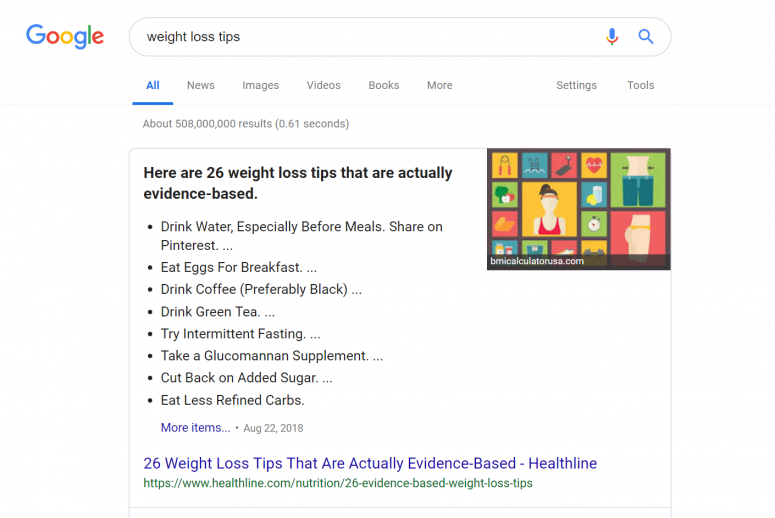The image is a screenshot of a Google search results page. The Google logo, featuring the iconic blue, red, yellow, and green colors, is prominently displayed in the upper left corner. Below the logo, the search bar shows that someone has queried "weight loss tips." The "All" tab is selected, highlighted in blue and underlined. The top search result is bold and black, stating, "Here are 26 weight loss tips that are actually evidence-based." Listed below the headline are several tips, including: "Drink water, especially before meals," "Eat eggs for breakfast," "Drink coffee, preferably black," "Drink green tea," "Try intermittent fasting," "Take a glucomannan supplement," "Cut back on added sugar," and "Reduce refined carbs."

In the upper right corner of the page, there is an image with a black border. This image is a collage featuring weight loss-related visuals, including a woman wearing a headband and tank top, appearing to exercise, a heart, a scale, and some exercise equipment.

At the bottom of the screenshot, another search result appears, with the headline "26 weight loss tips that are actually evidence-based" in purple text. Below this headline, the web address is displayed in green.